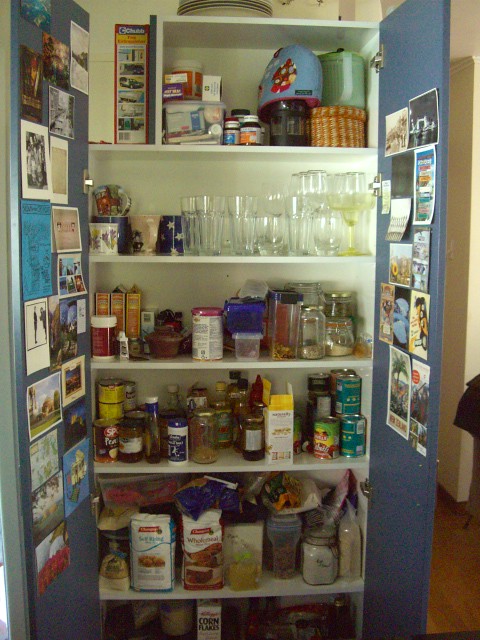The image depicts an open pantry cupboard that spans from the floor to about six or seven feet high. The pantry features two blue cabinet doors adorned with numerous postcards, pictures, and signs. Inside, there are six shelves, each meticulously organized:

1. **Bottom Shelf:** Partially visible, it holds a box of cornflakes and a jar.
2. **Second Shelf:** Contains large bags likely filled with ingredients such as flour or sugar, along with some jars.
3. **Third Shelf:** Stocked with canned goods and various jars.
4. **Fourth Shelf:** Holds an assortment of jars and boxes, possibly including rice.
5. **Fifth Shelf:** Lined with glasses, wine glasses, drinking glasses, and mugs.
6. **Top Shelf:** Shorter in width at about 75-80% of the pantry's span, it houses a small basket, some jars, and possibly some cereal.

The right side of the image provides a glimpse into the adjoining space of the house.